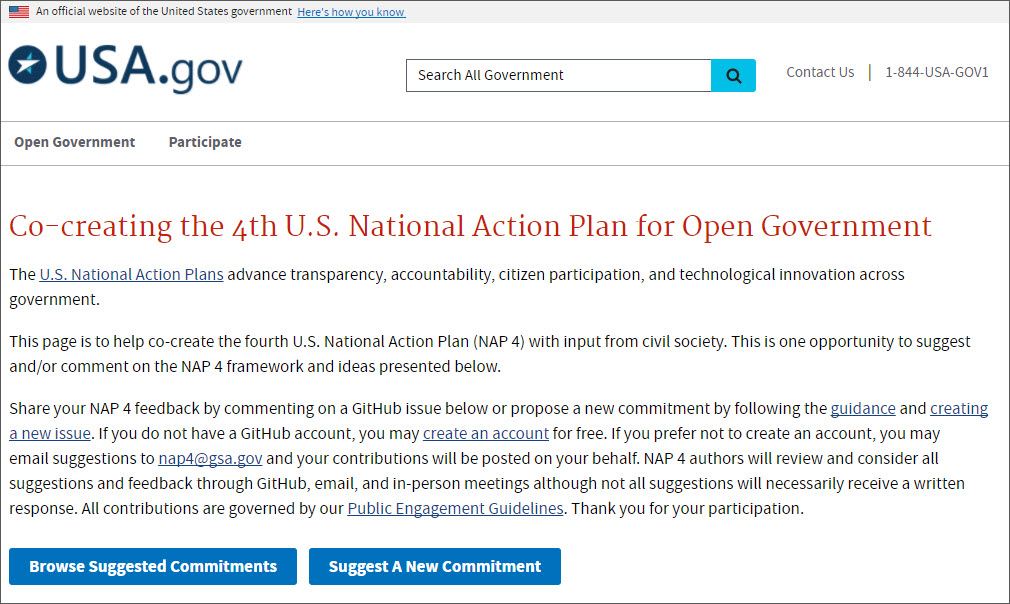In the top left corner, there is a small square image of the American flag. Adjacent to this image, text states "An official website of the United States government" with "Here's how you know" underlined in blue. Bold capital text "USA" followed by ".gov" appears next to a navy blue circle. To the right, there is a long search bar labeled "Search all government" with a blue search button at its end. Further right, small text reads "Contact Us" adjacent to a vertical dividing line and the phone number "1-844-USA-GOV-1."

Below this section, a box features the headings "Open Government" and "Participate." A bold red header follows, reading "Co-creating the Fourth U.S. National Action Plan for Open Government." "U.S. National Action Plans" is underlined in blue and introduces text explaining that these plans aim to advance transparency, accountability, citizen participation, and technological innovation across the government. Finally, there are two informational paragraphs, containing several key phrases underlined in blue: "Guidance," "Creating a new issue," "Create an account," "NAP4 at gsa.gov," and "Public engagement guidelines."